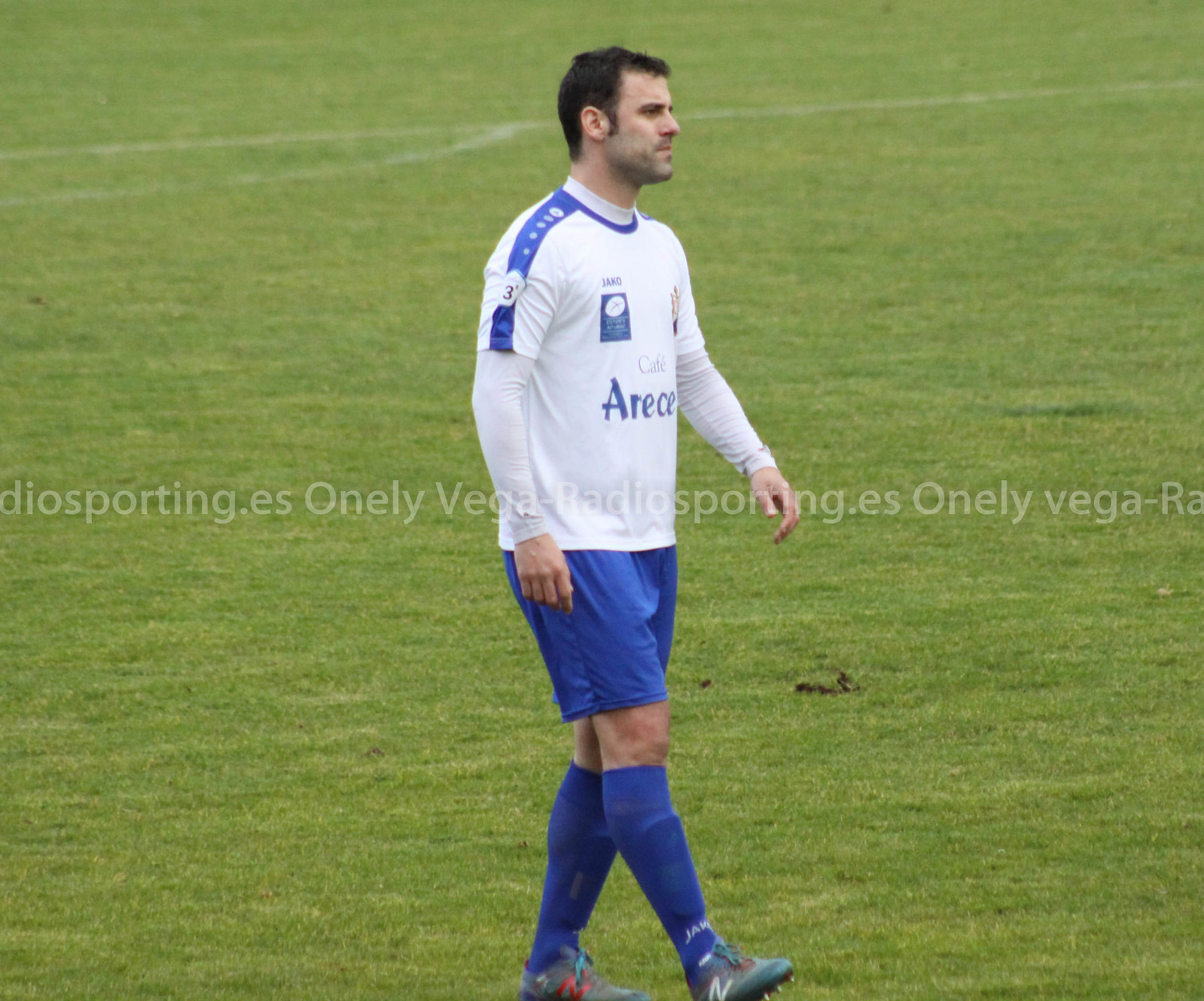In the middle of a vibrant green soccer field, an athlete stands alone, surrounded by white line markings that frame the scene. Wearing a white jersey with blue on the shoulders, blue shorts, blue socks, and muted blue shoes, he strikes a solemn pose, looking off to the right. The athlete has a fair complexion and black hair. His jersey features a partially visible logo that reads "Ares," along with blue and red accents and a number 3 on the shoulder. He appears to be making a subtle kicking motion with one foot. A faint watermark, "funlyvegassomething.es," is visible on the image, indicating the photographer or source of the photo.